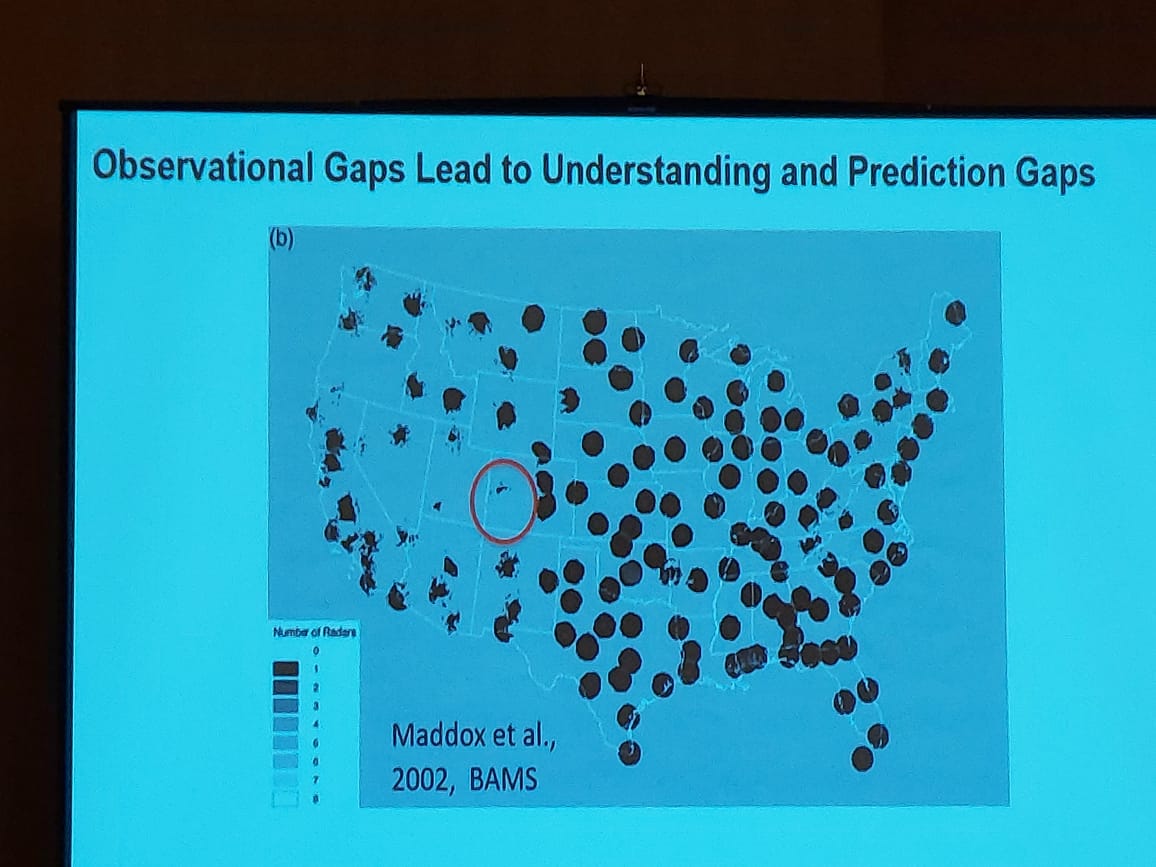The image is a photo of a presentation slide taken indoors, projected onto a large screen. The slide has an aqua blue background, and it prominently features the title "Observational Gaps Lead to Understanding and Prediction Gaps" in black letters at the top. Below the title, there is a large, somewhat unclear map of the United States with numerous black dots scattered across it. These dots denote different numbers of radars, with well-formed circular spots prevalent in the central and eastern parts of the country, while the western part has more irregular, stain-like spots. A specific region with very few radars is highlighted with a red circle. To the left of the map, there is a key indicating the number of radars: brown represents 1, dark brown also represents 1, light brown is 2, blue is 3, lighter blue is 4, and the lightest blue is 5, with each color corresponding to different levels of radar coverage. At the bottom of the slide, on the left-hand side, it says "number of readers or raters," and next to it, in black text, it reads "Maddox et al. 2002, BAMS."